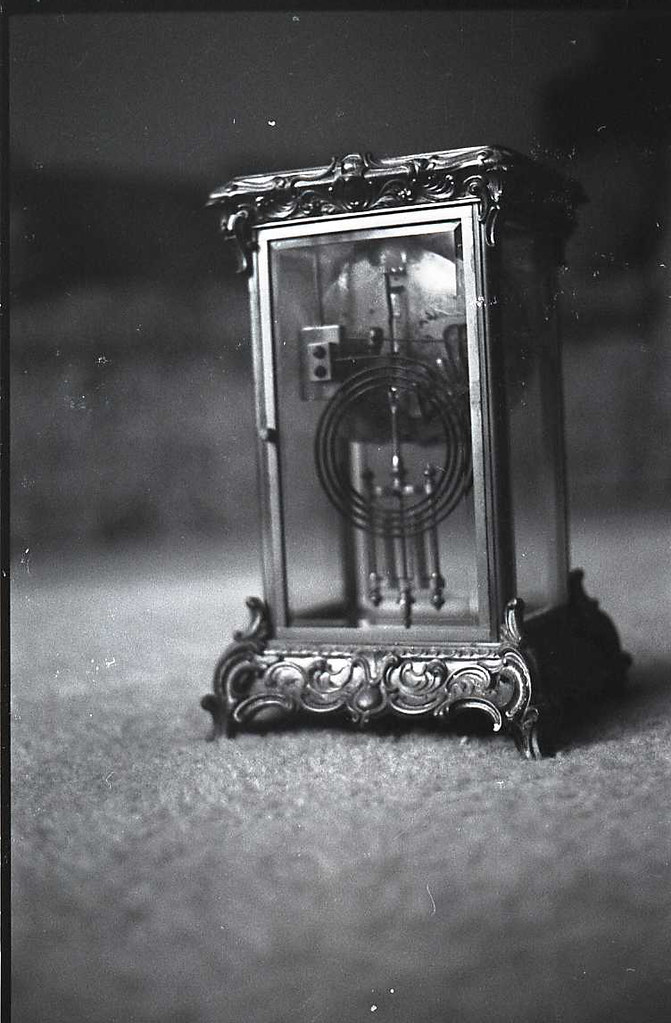In this photograph, we see the back view of a beautifully crafted, vintage pendulum alarm clock encased in beveled glass. The clock showcases intricate details, from the ornate top and bottom, complete with decorative feet, to the beveled door that grants access to the inner mechanics. The pendulum, situated at the bottom, is accompanied by three vertical weights that are a key part of the clock's functioning. The spring mechanism and inner workings of the clock are facing away from the viewer, highlighting the hammer poised to strike the spiral, creating the alarm sound. This elegant timepiece is placed on a speckled, vintage carpet, with a gray background that contrasts with the clock's craftsmanship, making the details stand out even more.